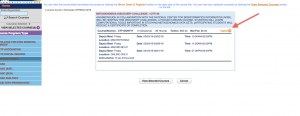In this screenshot of a website, the overall layout and text elements are largely unreadable due to the small size of the image. On the left side of the screenshot, there is a dark blue rectangle featuring red text. Directly below this, a gray section contains a search box. Further down, a purple rectangle with text is visible. Beneath this, there is a section with three blue rectangles containing text. This is followed by a darker blue rectangle. The next section comprises four blue rectangles with black text. To the right of these sections, at the very top of the image, there is a line of text in blue and orange. Below this line of text, a chart is displayed. The chart includes around four different labels at the top. Added onto this chart is a red arrow pointing to a word situated towards the right end of the top line.